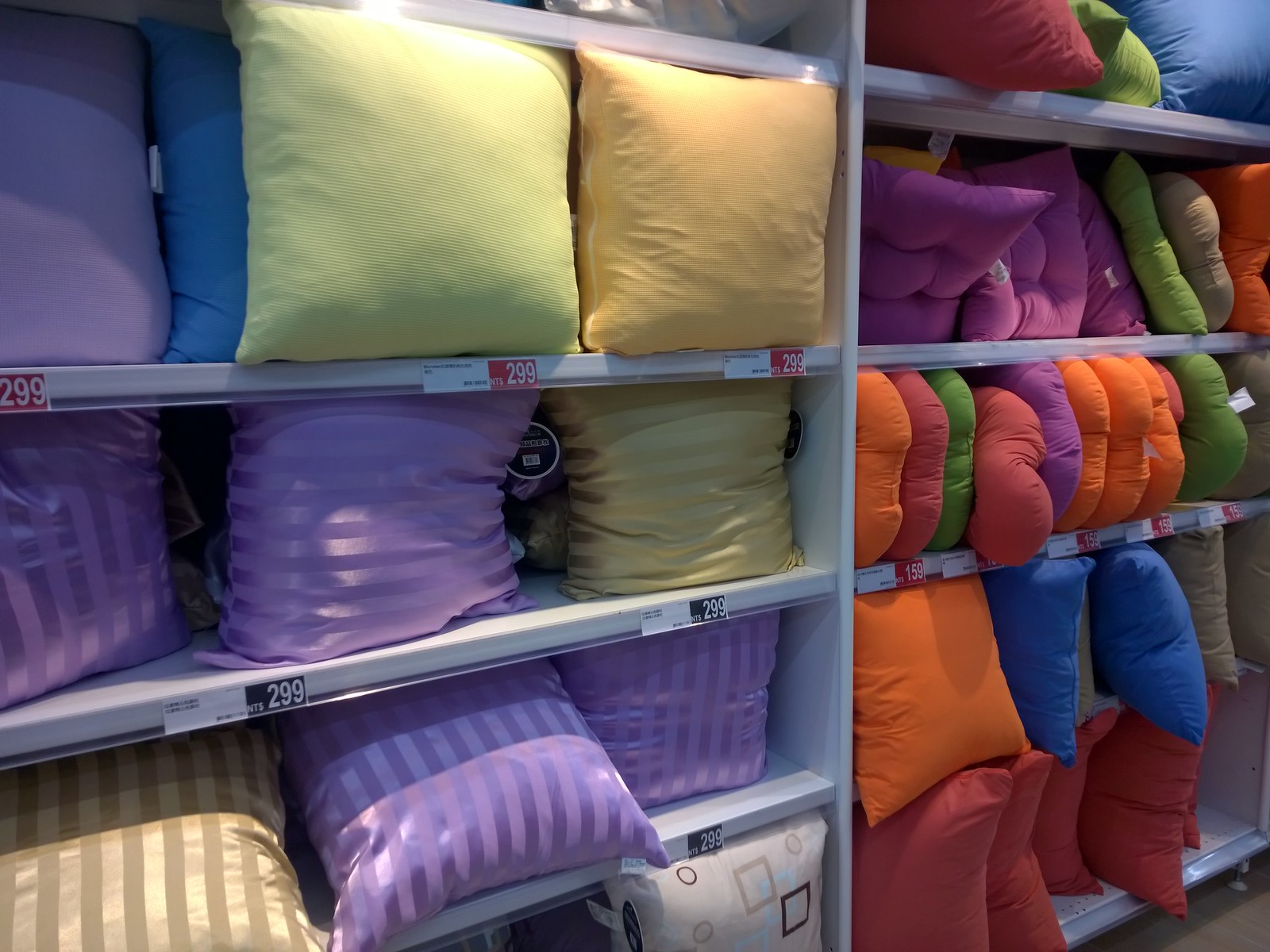This color photograph showcases a metal shelving display in a store, specifically arranged for showcasing a variety of pillows. The display is divided by a silver border at the center, separating the left and right sections. Each section contains multiple shelves filled with vibrant, stylish pillows.

On the left side, there are four visible shelves laden with large, fluffy pillows in shades of purple, blue, white, and a lighter yellow. Some of these pillows feature satiny stripes. Notably, each shelf on this side prominently displays a red price tag of $2.99. 

On the right side, there are five shelves, though only the bottom of the top shelf is visible, displaying pillows in red, green, and blue. Moving down, the next shelf exhibits pillows in colors like purple, green, white, and brown, neatly arranged with their edges facing outward. The subsequent shelf features pillows in plain designs, including shades of green, pink, orange, and purple, while the bottom shelf is uniformly arranged with dark red pillows. Price tags on this side occasionally show $1.59 in red or blue areas.

The entire shelving fixture is a light grey color, and the floor beneath it is brown. One cushion in the bottom middle of the picture sports a beige background with a brown and blue abstract or square design, adding to the diversity of designs and colors on display. The comprehensive arrangement not only highlights the various colors but also the different designs and textures of the pillows, making for an eye-catching retail presentation.